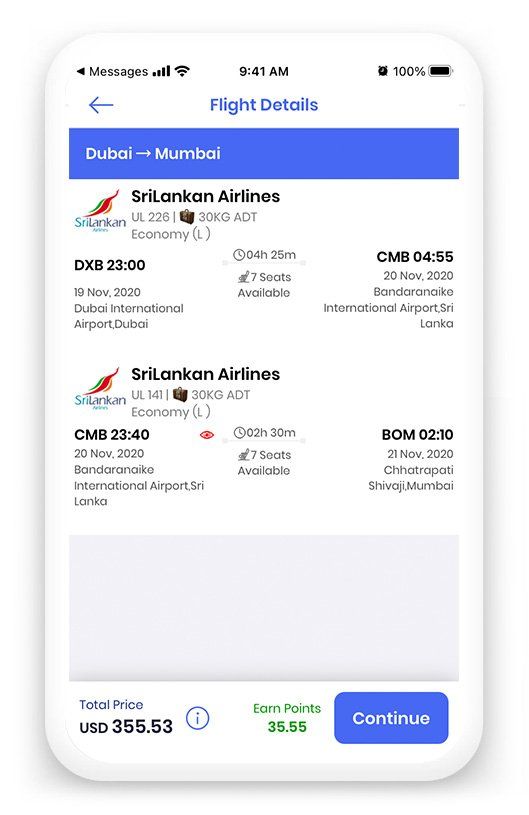Certainly! Here's a refined and detailed caption for the image you described:

---

**Image Caption**

This screenshot, likely from an iPhone, displays detailed flight information with a predominantly white interface. At the top of the screen, status indicators show "Messages," a strong Wi-Fi signal, the time (9:41 AM), and a fully charged battery icon.

Below this, a blue text header reads "Flight Details," accompanied by a left-pointing arrow. The main section features a blue rectangular banner with "Dubai to Mumbai" prominently displayed, followed by comprehensive airline information. The airlines identified is Sierra Lincoln Airlines, denoted with its logo.

Key flight details include:
- **Flight Number:** UL-226 (Economy Class)
- **Departure:** Dubai International Airport (DXB), November 19th at 23:00
- **Duration:** 4 hours, 25 minutes
- **Seats Available:** 7
- **Arrival:** Bandaranaike International Airport (CMB), Sri Lanka, November 20th at 04:55

The return flight information is also provided:
- **Flight Number:** UL-141 (Economy Class)
- **Departure:** Bandaranaike International Airport (CMB), November 20th at 23:40
- **Duration:** 2 hours, 30 minutes
- **Seats Available:** 7
- **Arrival:** Chhatrapati Shivaji Maharaj International Airport (BOM), Mumbai, November 21st at 02:10

At the bottom portion of the screen, a blank white rectangular box is present, followed by the total price of the journey, listed as USD $355.50. There is also an information icon next to the price. Additionally, air points accrued amount to $35.55, and a "Continue" button is provided for further action.

---

This caption captures all the essential details presented in the image, formatted in a concise and organized manner.